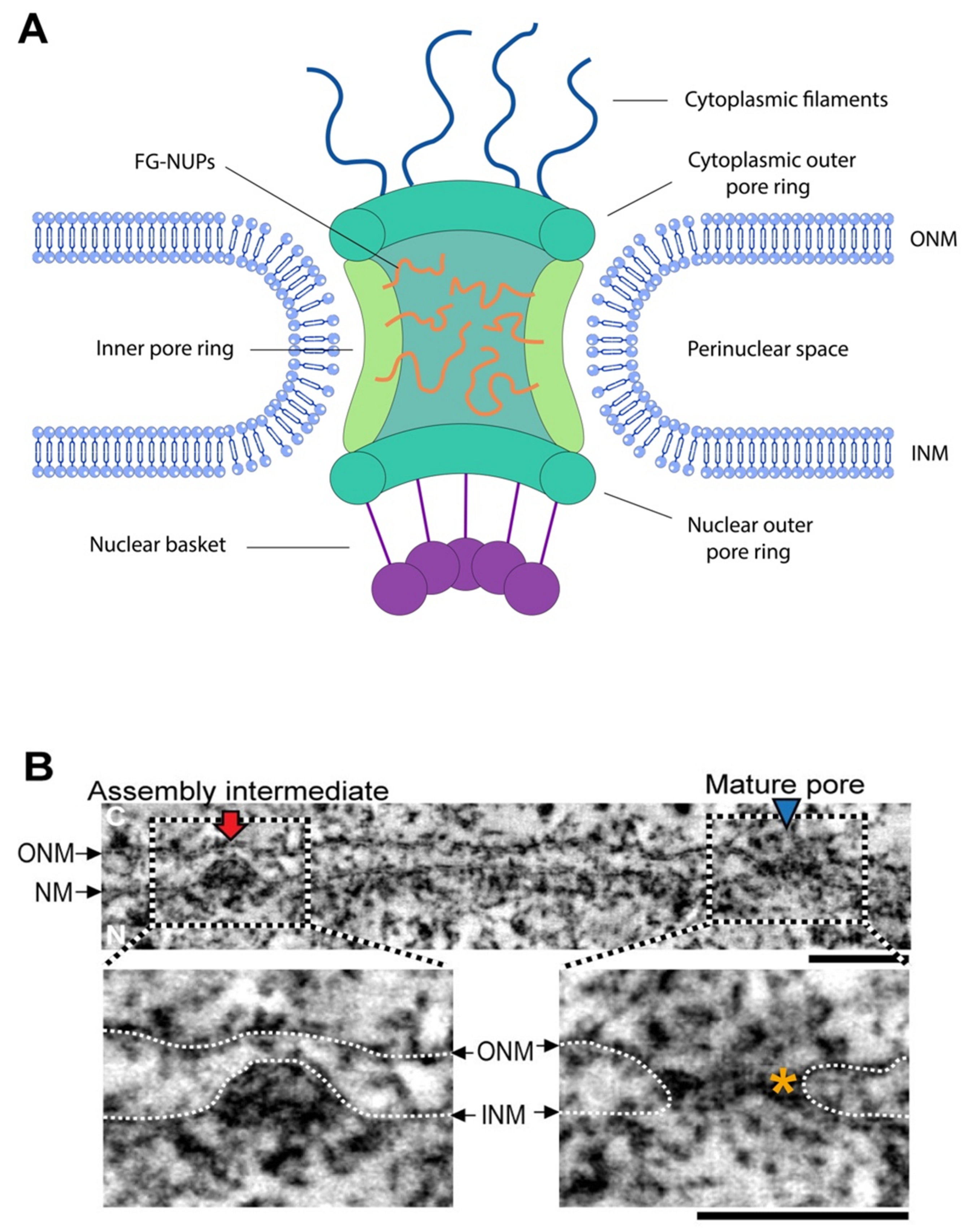The image presents a detailed representation of the structure of the nuclear pore complex depicted in two sections, labeled A and B. The upper section (A) features a schematic illustration of the nuclear pore, a large protein complex that spans the nuclear envelope. Central to this illustration is a green structure with embedded orange FG-NUPS filaments. Extending from the top of this green core are four blue cytoplasmic filaments, while the bottom part is anchored by purple lines ending in purple circles, indicative of the nuclear basket on the nuclear side of the pore. The illustration also highlights the perinuclear space, cytoplasmic outer pore ring, nuclear outer pore ring, and inner pore ring with horseshoe-shaped structures on both sides.

The lower section (B) comprises three black-and-white electron microscope images, each accompanied by descriptive text and arrows. These images likely demonstrate various stages of nuclear pore assembly, identified by red and blue arrows pointing to intermediate and mature pores, respectively. Annotations such as ONM (outer nuclear membrane), INM (inner nuclear membrane), and NM (nuclear membrane) provide additional context to the microscopic visual data. The overall presentation combines graphical and photographic techniques to elucidate both the structural components and the assembly process of the nuclear pore complex, offering a comprehensive educational resource for those familiar with cellular biology.